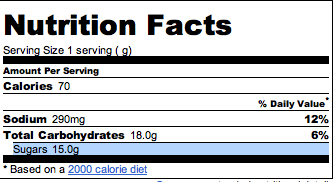This image is a detailed view of a Nutritional Facts label, typically found on the back of food packaging. The label itself appears to be a digital version, devoid of any product context. At the top, 'Nutrition Facts' is prominently displayed in bold print. Directly below, in smaller text, it specifies the serving size as one serving. A horizontal black border separates this from the next section, which lists the Amount Per Serving: Calories are 70. Subsequent sections are delineated by small borders indicating various nutritional values. Sodium is listed at 290 milligrams, accounting for 12% of the daily value. Total carbohydrates are 18 grams, representing 6% of the daily value, with sugars listed at 15 grams in blue highlight. The overall layout is enclosed within a thin border, noting that these values are based on a 2,000 calorie diet.